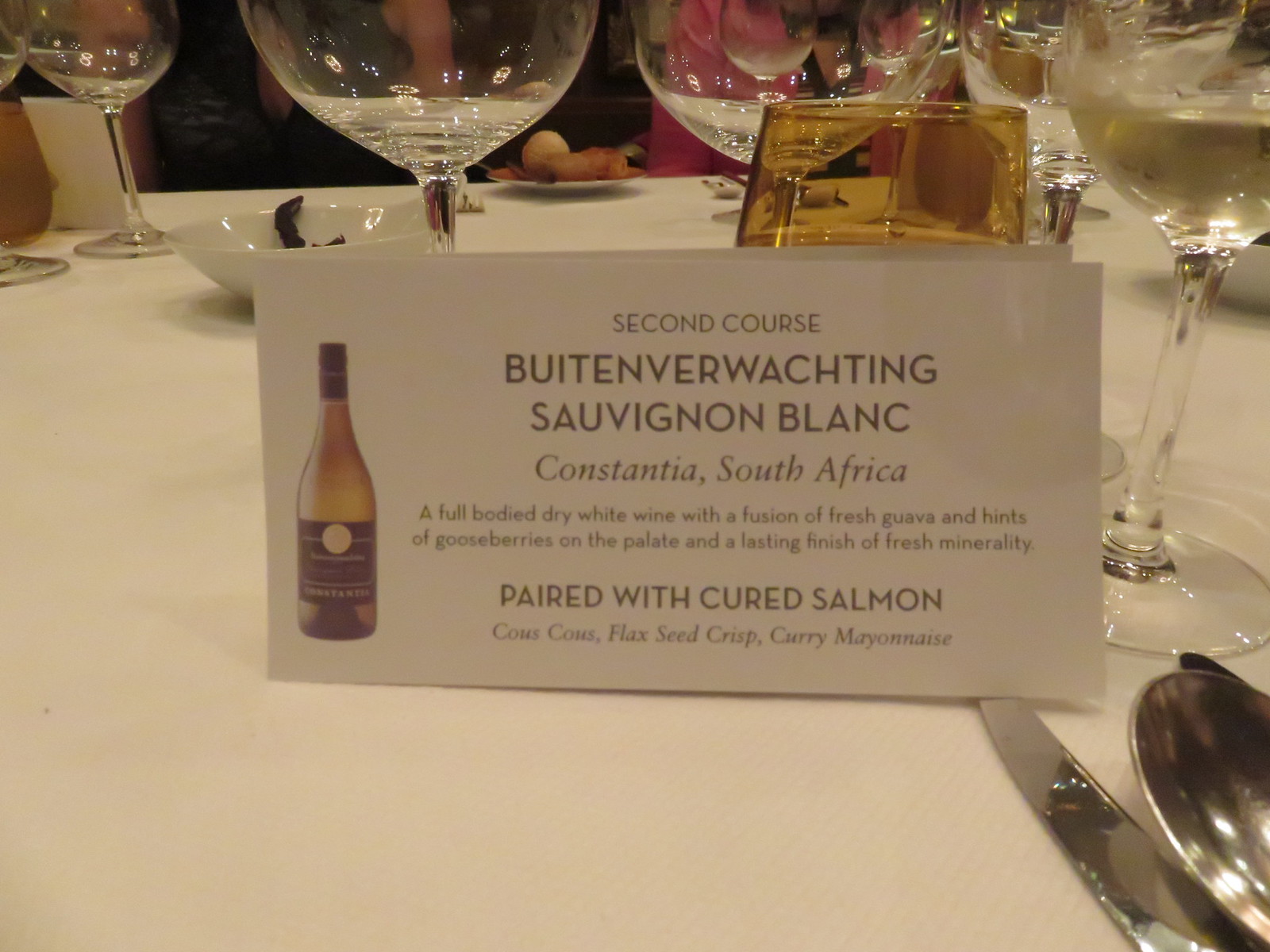The image depicts an elegant table setting at what appears to be a formal event or a sophisticated restaurant. The setting features a large white table covered with a white tablecloth. The focal point is a white placard positioned at the center of the table, bordered by wine glasses and silverware. The placard is a landscape-oriented rectangle with black text on the right side and an image of a green wine bottle on the left. The text reads "Second Course" at the top, followed by "Wittenverwachten Sauvignon Blanc." It also mentions "Constantia, South Africa," describing the wine as "a full-bodied dry white wine with a fusion of fresh guava and hints of gooseberry on the palate, and a lasting finish of fresh minerality." Below that, it indicates the wine is "Paired with cured salmon, couscous, flaxseed crisp, curry mayonnaise." The setting is further detailed with silver cutlery on the lower right and an assortment of white bowls, adding to the formal dining experience. The color scheme includes white, brown, black, red, pink, tan, and silver, contributing to the overall sophisticated ambiance of the setting.